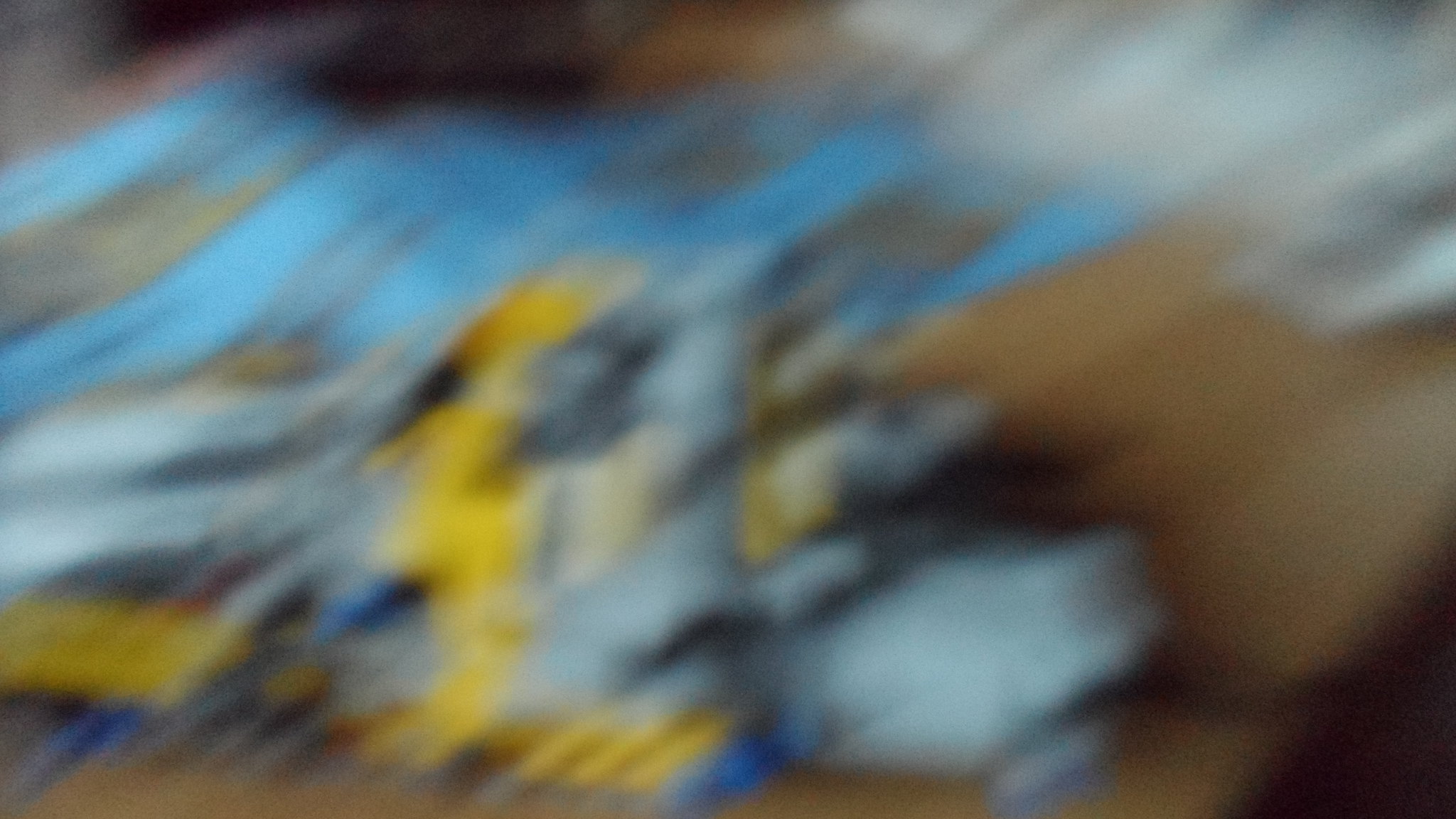The photograph is a very blurry, low-resolution image in landscape format, making it difficult to discern any specific details or objects. It appears to be an abstract mix of colors—predominantly shades of blue, gray, white, yellow, tan, brown, and black. The orientation of the blur suggests that the camera moved diagonally from either bottom left to top right or top right to bottom left, creating a slanted grain effect. Despite the blurriness, the colors and the possible brown background suggest an object, possibly held by someone, photographed out of focus on a desk or table. There is no text or any clear indication of what the image is supposed to represent.